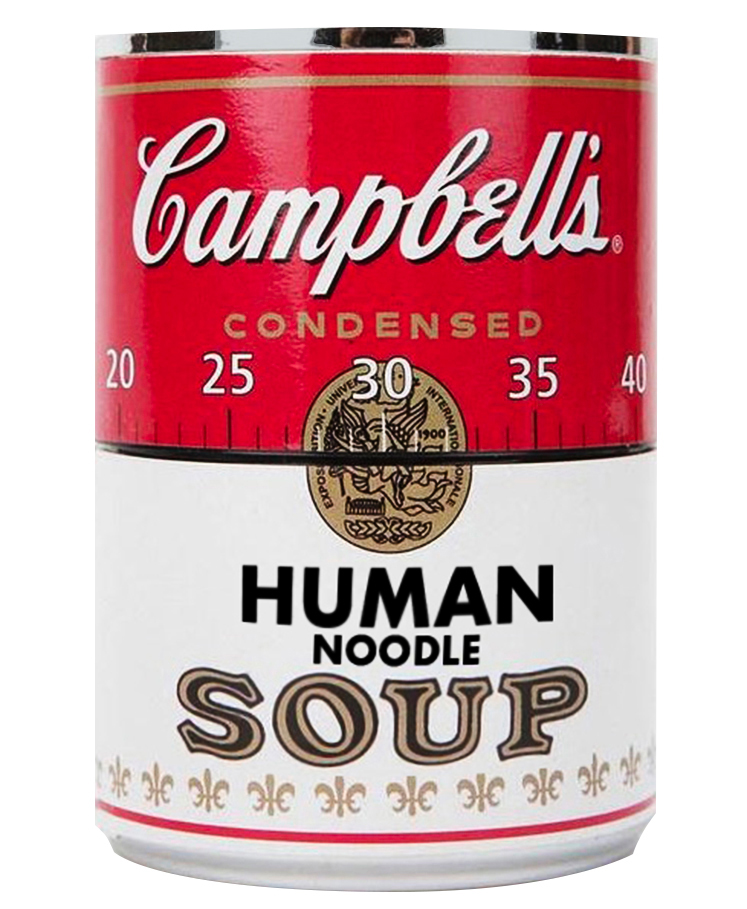This detailed, computer-generated image depicts a can of Campbell's Condensed Human Noodle Soup, combining features seen in classic Campbell's soup can designs with a whimsical twist. The upper portion of the can features a red background with the iconic "Campbell's" written in white cursive text. Below this, in a goldish color, is the word "Condensed." A ruler-like measurement scale runs horizontally across the can with numbers 20, 25, 30, 35, and 40, separated by small notches. The center of the label displays a gold circle with an indistinct emblem, possibly reading "University," with a black vertical line running through it. Beneath this, the words "Human Noodle" are prominently displayed in black text on a white background, while the word "Soup" is rendered in a mix of black and brown. The bottom section of the can features brownish-golden decorative designs, ending with a red horizontal line that neatly divides the label from the silver-metal base of the can.